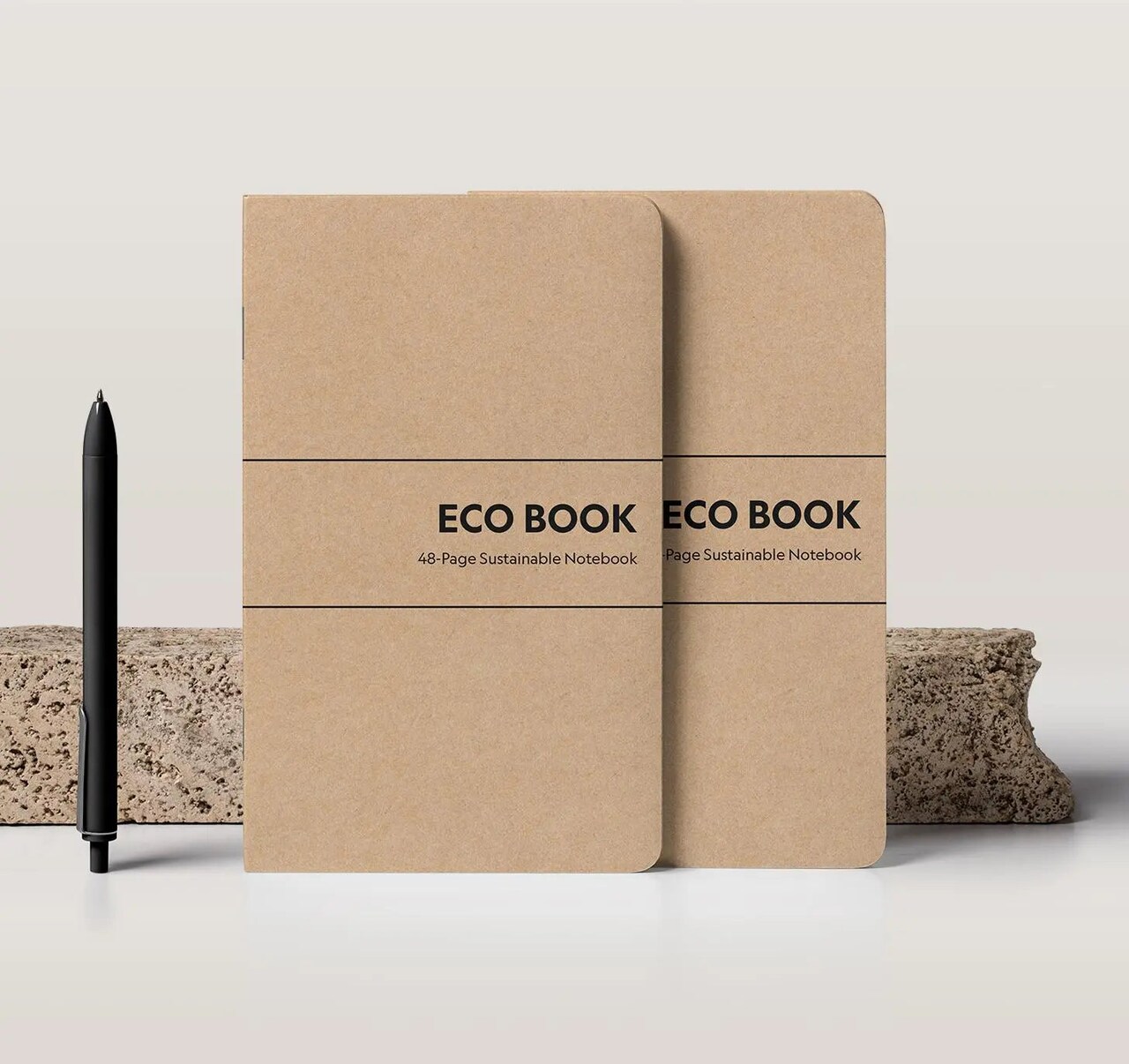The image features two eco-friendly, cardboard-finished notebooks arranged one on top of the other, on a white table or countertop against a white background. The notebooks have two horizontal black lines forming a rectangular outline in the center. Inside this outlined area, in bold, black, capital letters, it reads "ECO BOOK," and below that, the text "48 PAGE SUSTAINABLE NOTEBOOK" is displayed. To the left of the notebooks, a black ink pen stands upright on its clicker. Behind the notebooks, there is a rectangular piece of rough, beige stone, displaying visible pores and a broken right edge. The overall scene emphasizes a minimalist and eco-conscious aesthetic.